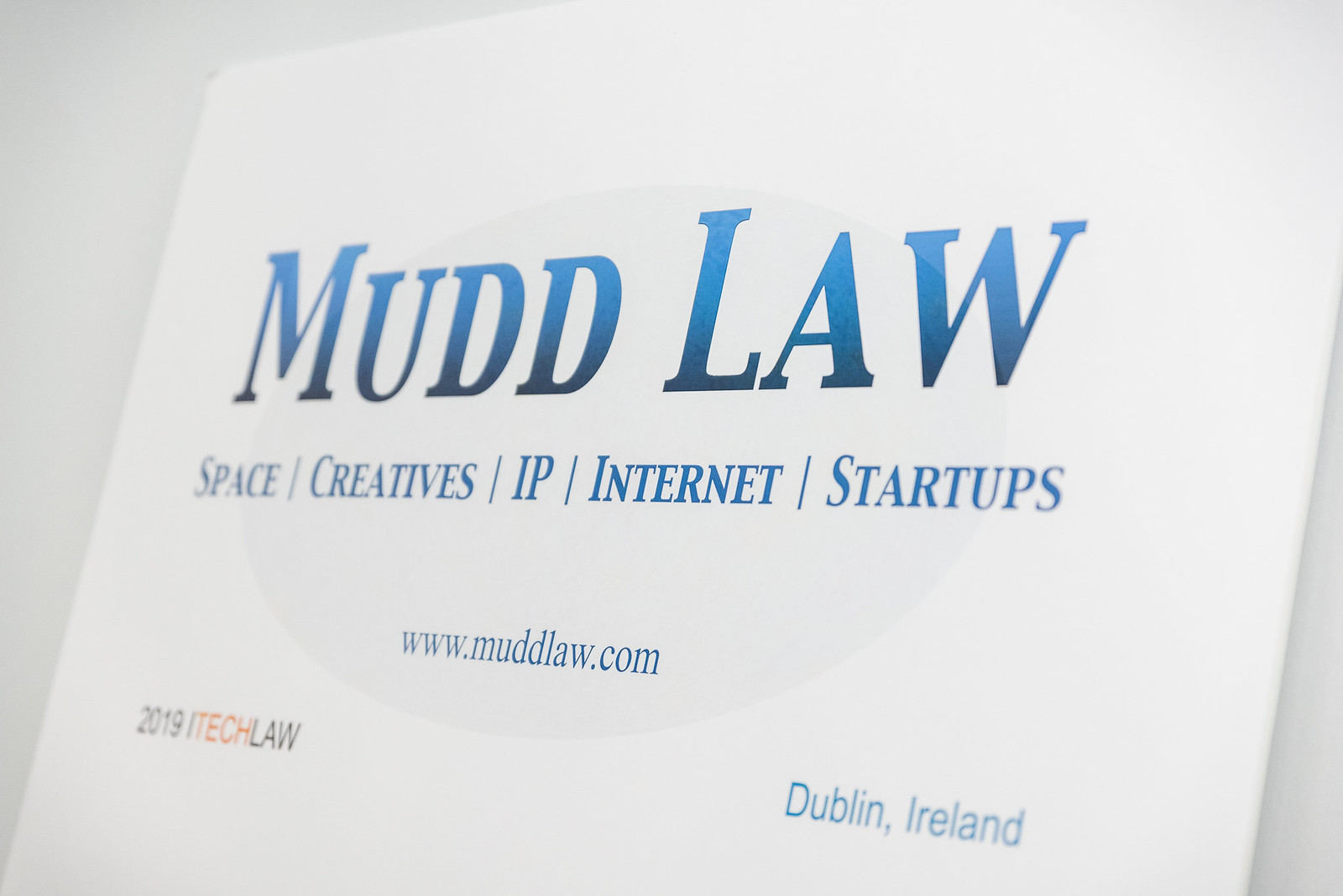This image is a close-up photograph of a white business card, taken at an angle. The card features a subtle gray oval design in the center. In large blue gradient letters at the top, it reads "Mud Law" with "Mud" spelled with two D's. Beneath this, separated by short vertical lines, are the words "Space, Creatives, IP, Internet, Startups" in smaller blue letters. At the very bottom, also in blue, is the website URL "www.mudlaw.com." In the bottom left corner, it states "2019 iTech Law," and in the bottom right, it says "Dublin, Ireland." The card has a clean, minimalistic design, set against an off-white background.